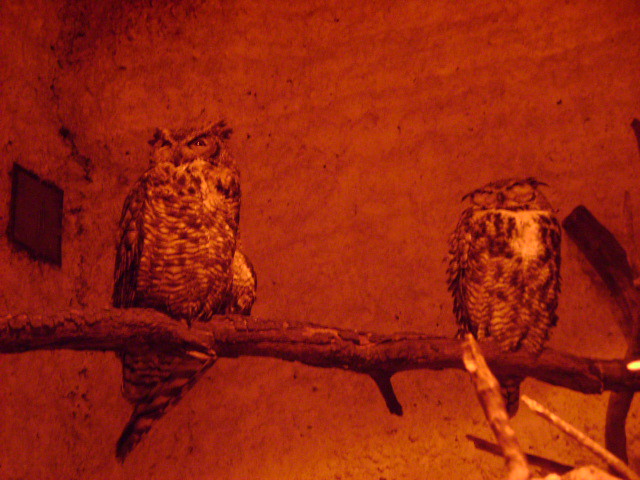The photograph captures two owls perched on a detailed, textured tree branch against an old stone building, giving the impression of a fort setting. The image is dominated by a washed red hue, possibly due to a red filter or dusk lighting, which tints the owls' feathers in shades of red and orange with flecks of black. The larger owl, positioned on the left with open eyes, has its head slightly crooked to the left and its ears flattened. The smaller owl on the right, with its eyes closed, shares a similar head tilt. Both owls' tails hang below the branch, which extends horizontally across the frame. The backdrop features a light yellow to tan wall with a square object—potentially a window or a vent—behind the larger owl. Additional branches appear in the foreground at the bottom right. The overall scene, devoid of textual elements, evokes a serene yet eerie atmosphere, enhanced by the stark contrasts and rich details within the image.